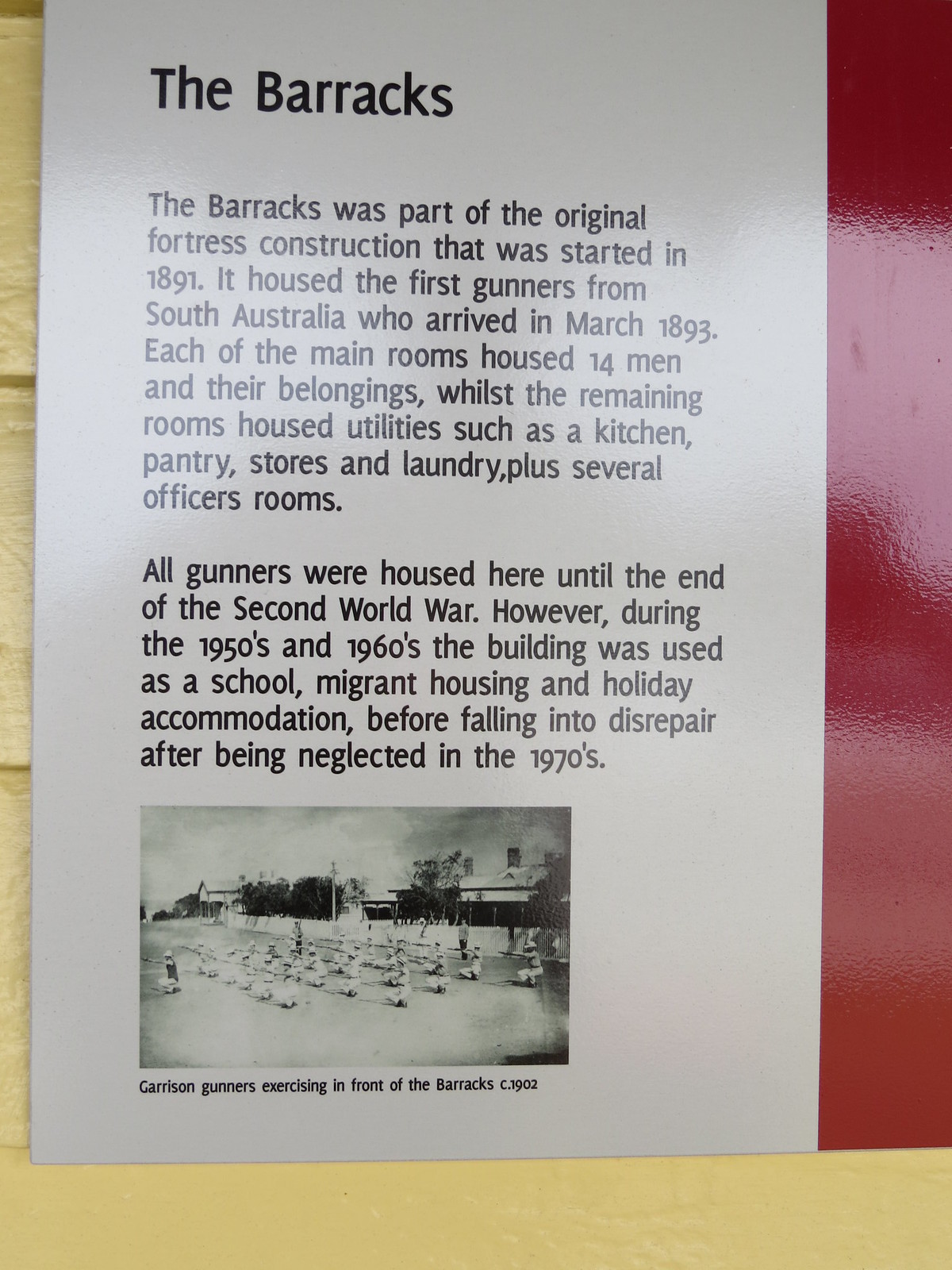The photograph captures a museum sign affixed to a wall, providing historical information. The sign is rectangular with a stark white background, and it’s divided into sections of text and imagery. The top of the sign features the bold title, "The Barracks," followed by two paragraphs detailing the history of the barracks. It explains that the barracks were part of the original fortress construction initiated in 1891, housing the first gunners from South Australia who arrived in March 1893. The text elaborates that the main rooms accommodated 14 men and their belongings, with other rooms designated for utilities such as a kitchen, pantry, stores, and laundry, as well as officers' rooms. The barracks served this purpose until the end of the Second World War, after which it was repurposed in the 1950s and 1960s for use as a school, migrant housing, and holiday accommodation, later falling into disrepair in the 1970s. Below the text, there is a rectangular, black-and-white photograph depicting several individuals engaged in a military drill in front of the barracks. The caption under the photograph reads, "Garrison Gunners Exercising in front of Barracks C-1902." The wall to which the sign is attached has a cream hue while the right side is painted red.